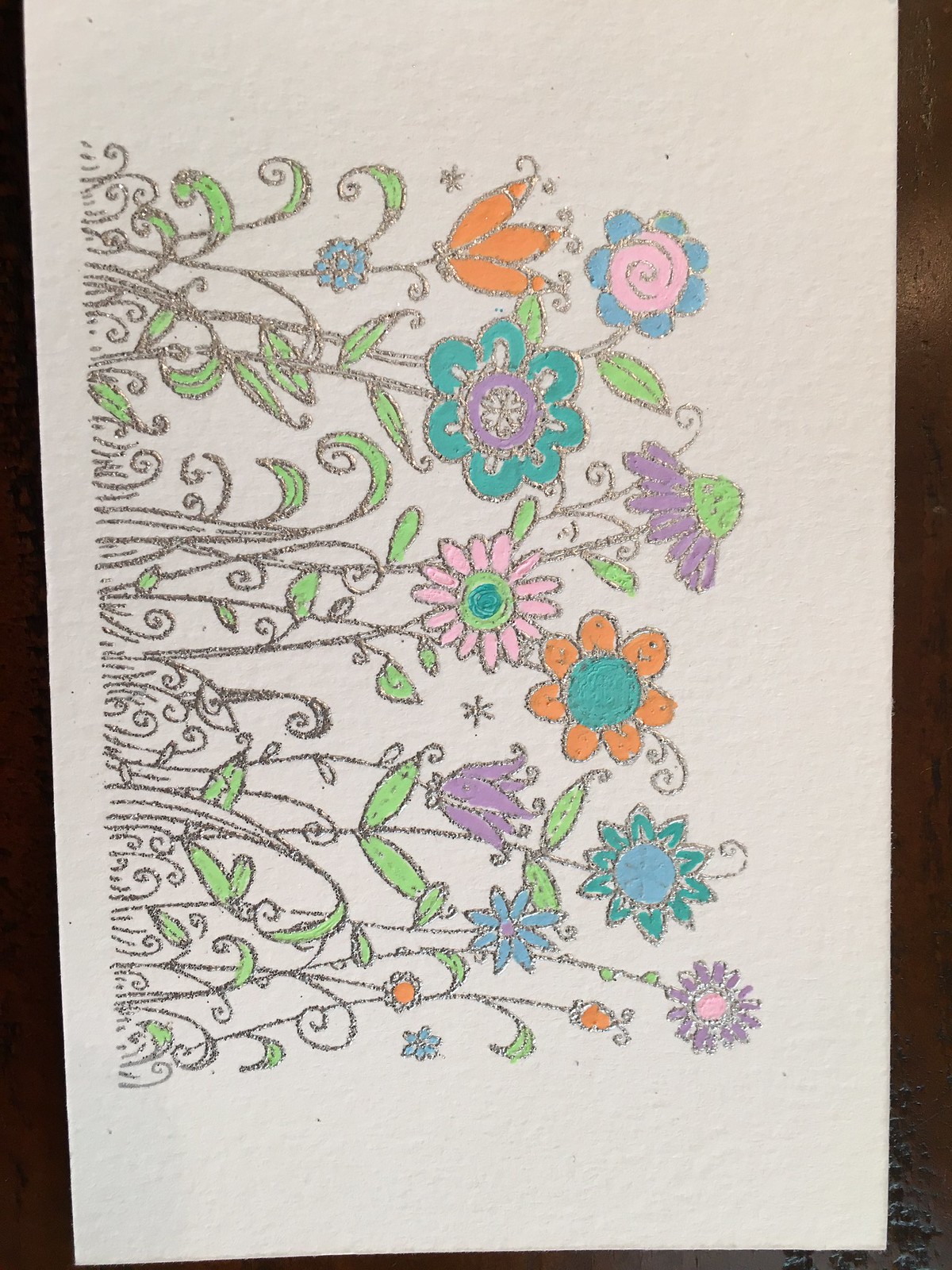A vibrant, hand-painted floral image on a white canvas is artfully turned on its side, offering a unique perspective. The flowers, depicted in an array of bright colors including pink, purple, blue, orange, and aquamarine, appear to be growing horizontally from a grassy texture at the base of the painting. The light green leaves complement the vivid blooms, creating a striking contrast. This enchanting composition is set against a dark brown wooden tabletop, enhancing the visual appeal of the artwork.